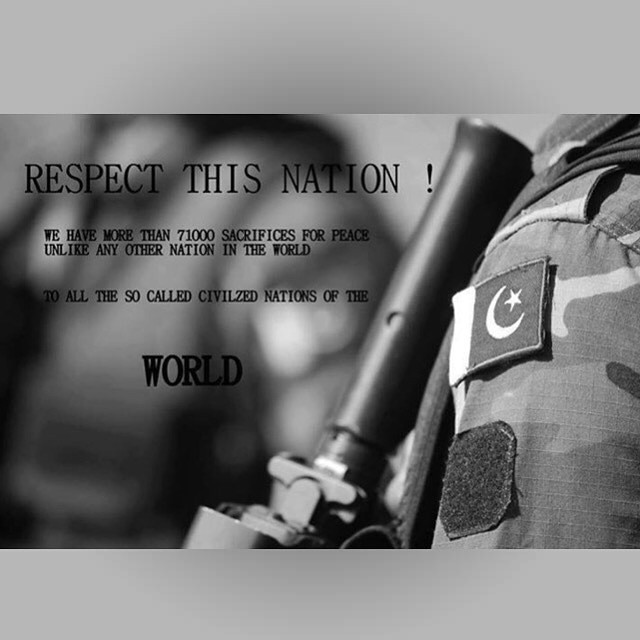The poster features a grayscale image predominantly in shades of black, white, and gray. At the center, framed by two horizontal gray borders at the top and bottom, is bold, black text in all capitals: "RESPECT THIS NATION!" Beneath it, also in black capital letters but smaller, it reads: "We have more than 71,000 sacrifices for peace, unlike any other nation in the world. To all the so-called civilized nations of the world." The imagery includes a zoomed-in view of a person in a camouflage military uniform, with only the top of their shoulder and part of their chest visible. Protruding against their chest is what appears to be a gun barrel. On the right shoulder of the uniform, a patch featuring the Russian flag with a star and moon emblem is visible. The image background is intentionally blurred, emphasizing the foreground elements and the impactful message intended for social media dissemination.